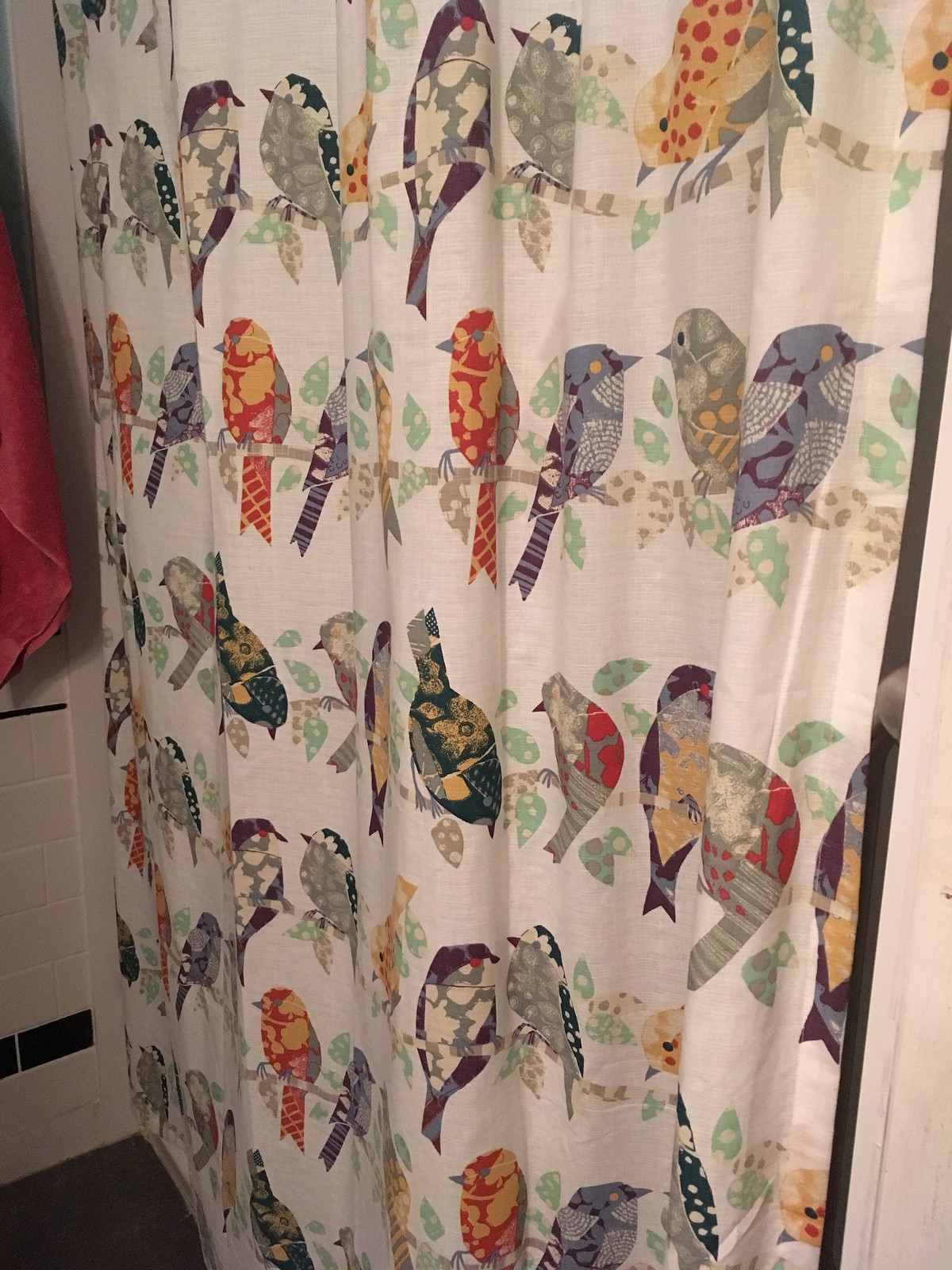In this well-lit, indoor color photograph of a bathroom, the central focus is a shower curtain adorned with artistic bird designs. The curtain, which extends from beyond the top of the visible frame to the dark brown floor, features a series of horizontal branches on which a variety of vibrantly colored birds are perched. The birds, depicted in non-realistic, pastel tones, include hues of brown, green, beige, light blues, oranges, yellows, and golds. The backdrop of the curtain is a light beige or very light tan, providing a subtle contrast to the detailed bird illustrations. To the left of the curtain, a beige tiled wall is bordered with brown, while a glimpse of dark brown flooring is visible at the bottom. An orange terry top or towel hangs nearby. The right side of the image shows a hint of a white wall. In the upper left corner, a portion of a pinkish towel is visible, suggesting the presence of a towel rack. The image captures a serene, earthy aesthetic with its natural tones and detailed decor.